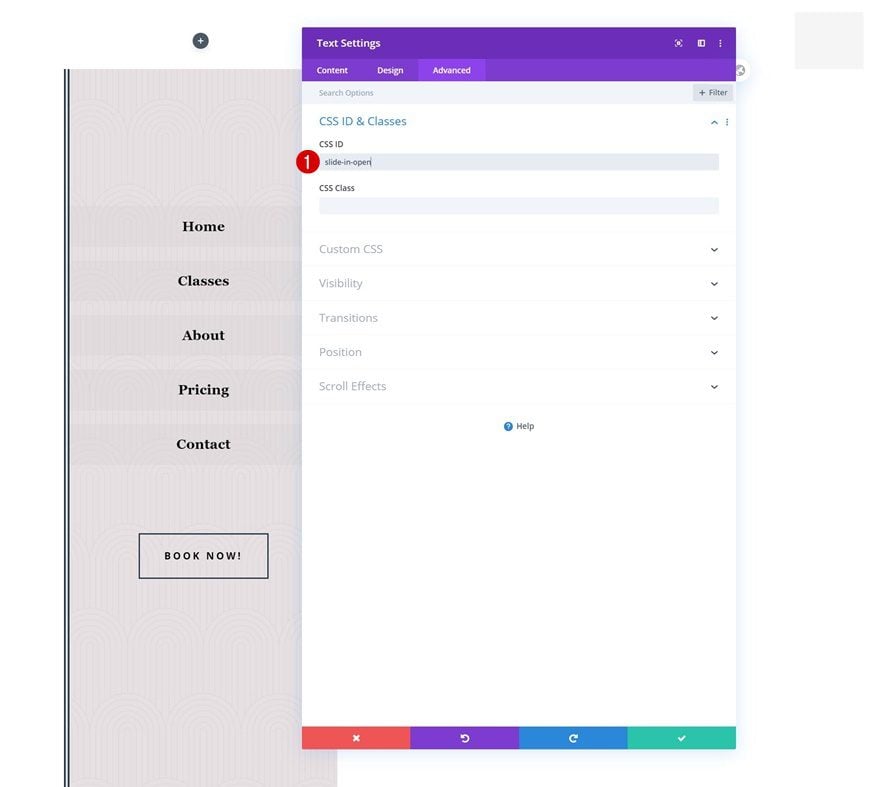A computer or mobile screen displays a user interface with multiple sections and menus. The layout is relatively wide, with a side navigation menu featuring options such as Home, Classes, About, Pricing, and Contact. These menu items are each styled in gray and black text but do not appear to be actively selected as none are highlighted or darkened. Below this menu is a prominent "Book Now" button.

At the top of the main interface section, there is another toolbar labeled "Test Settings". This toolbar includes three buttons: Content, Design, and Advanced, with the Advanced button being actively selected. The Advanced settings section provides options for CSS ID and Classes, where the CSS ID is identified as "slide to open" with a numeric designation of one (1). The classes section appears slightly darker than other text fields, indicating it's available for interaction.

Further down, there is a list of inactive, lighter gray options: Custom, Visibility, Transitions, Position, and Scroll Effects, implying these settings are not currently in use. Below these options, there is a center-justified help icon in a blue circle and accompanied by a question mark symbol.

At the bottom of the screen, a series of control icons are present, including 'X' for closing, back, forward, and an unidentified green button, which is not clearly labeled.

This interface appears to be a part of a more extensive web or app design tool, offering a variety of customizable settings for advanced users.